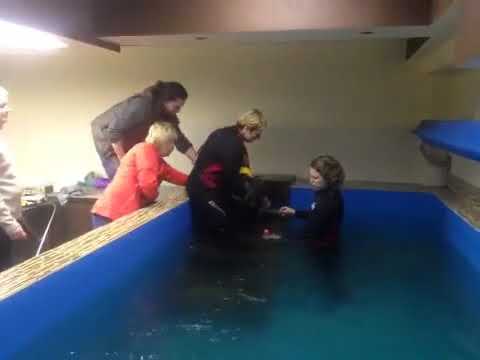In this square, somewhat blurry image, a central rectangular tub with raised wooden sides filled with water is the main focal point. Inside the tub, the interior appears blue and contains two women. One woman is partially immersed in the water, wearing a brown shirt and exhibiting short, curly brown hair. She has her hands extended in front of her, seemingly interacting with the other woman. The second woman, leaning over and engaging with the first, has short blonde hair and is dressed in a black outfit with pink and yellow accents. Surrounding the tub, a few other people are present. To the right, a woman in a long-sleeved red or orange jacket and another in a gray long-sleeve top with brown hair are visible. On the far left, partially captured, is another individual wearing a long-sleeved brown shirt. The background walls of the room appear white but might be ivory or beige, contributing to the indoor setting, which suggests a possible medical environment. Despite the varied lighting and color hues, the focus remains on the tub and the interactions within and around it.